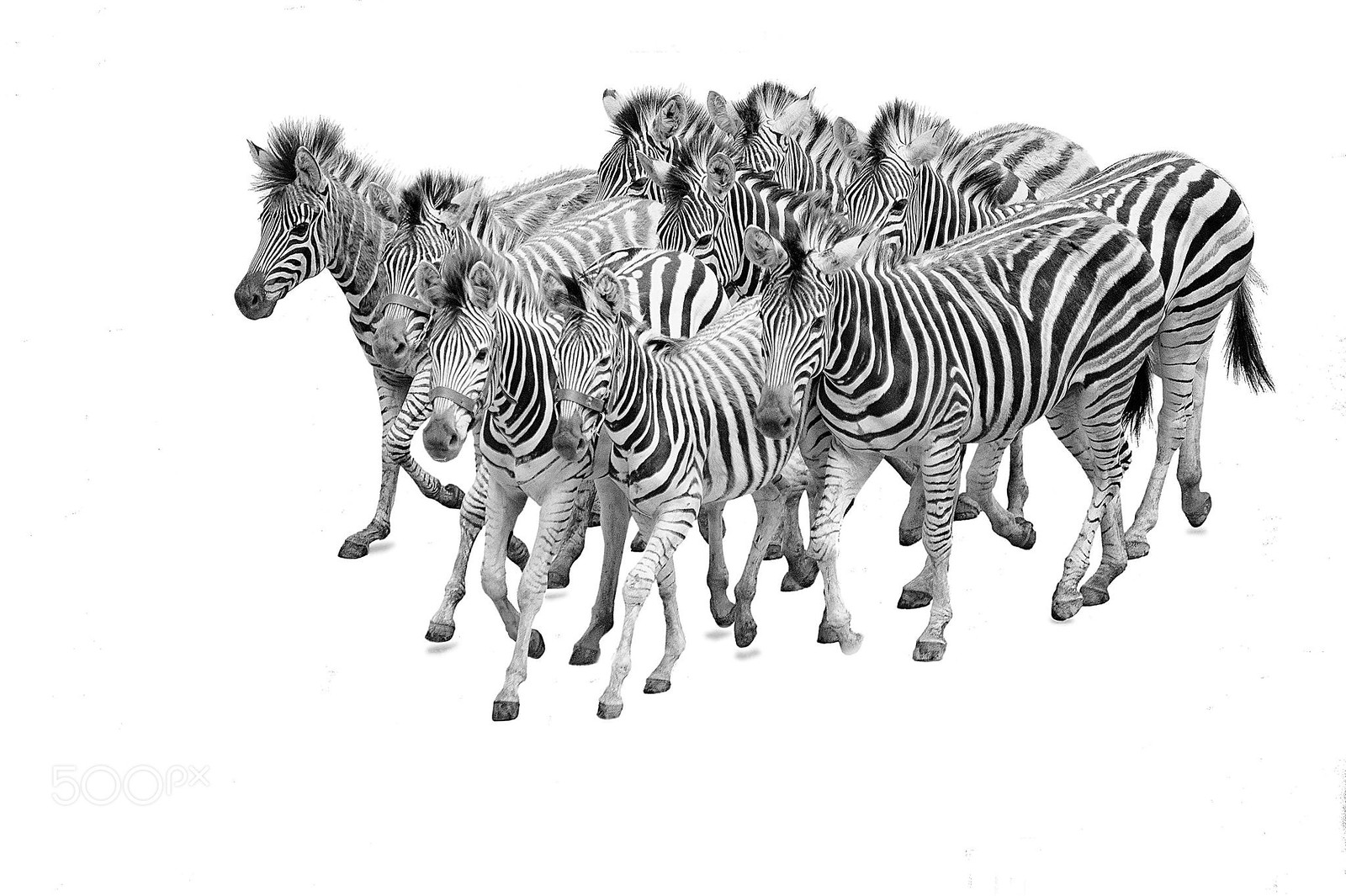The image features a digitally altered, black-and-white photograph of approximately nine zebras, arranged head-to-toe, facing diagonally from the upper right to the lower left corner. The background has been completely whited out. The zebras are closely packed together, creating a uniform line with their heads mostly facing forward. The smaller zebras at the front, likely younger ones, are distinguished by harnesses on their noses, whereas the rest are unadorned. This composite image gives the impression of a synchronized movement in unison, presenting a striking visual of this iconic African species.